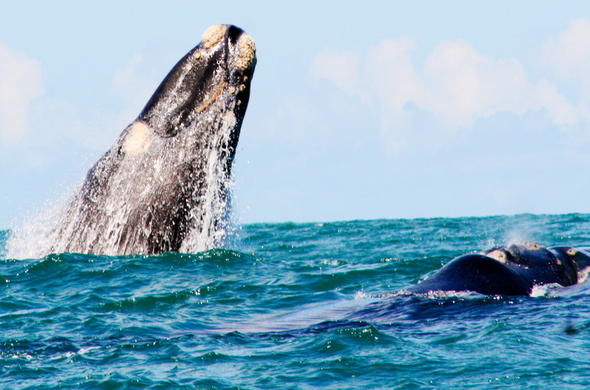The photograph captures a dramatic scene in the ocean, predominantly showcasing a towering breaching whale on the left side. This colossal marine mammal, described as a grey or blue whale, emerges almost vertically from the water with about a third of its body exposed. The whale's skin is primarily dark gray to black with patches of lighter colors, including some white or light tan areas, especially around its mouth, which is peppered with barnacles or other growths. As the whale ascends, water cascades off its body in a white frothy display, contrasting sharply with the deep blue and green shades of the ocean.

On the right side of the photograph, another large sea creature, possibly another whale, is visible. This figure, identified as dark blue in color, appears to be swimming or floating, though its exact nature is ambiguous. The serene sky above is a light blue adorned with scattered white, fluffy clouds, completing the picturesque maritime vista. 

This detailed description melds common observations about the breaching whale, its coloration, the cascading water, and the expansive ocean and sky, creating a vivid representation of the dynamic and vibrant seascape.